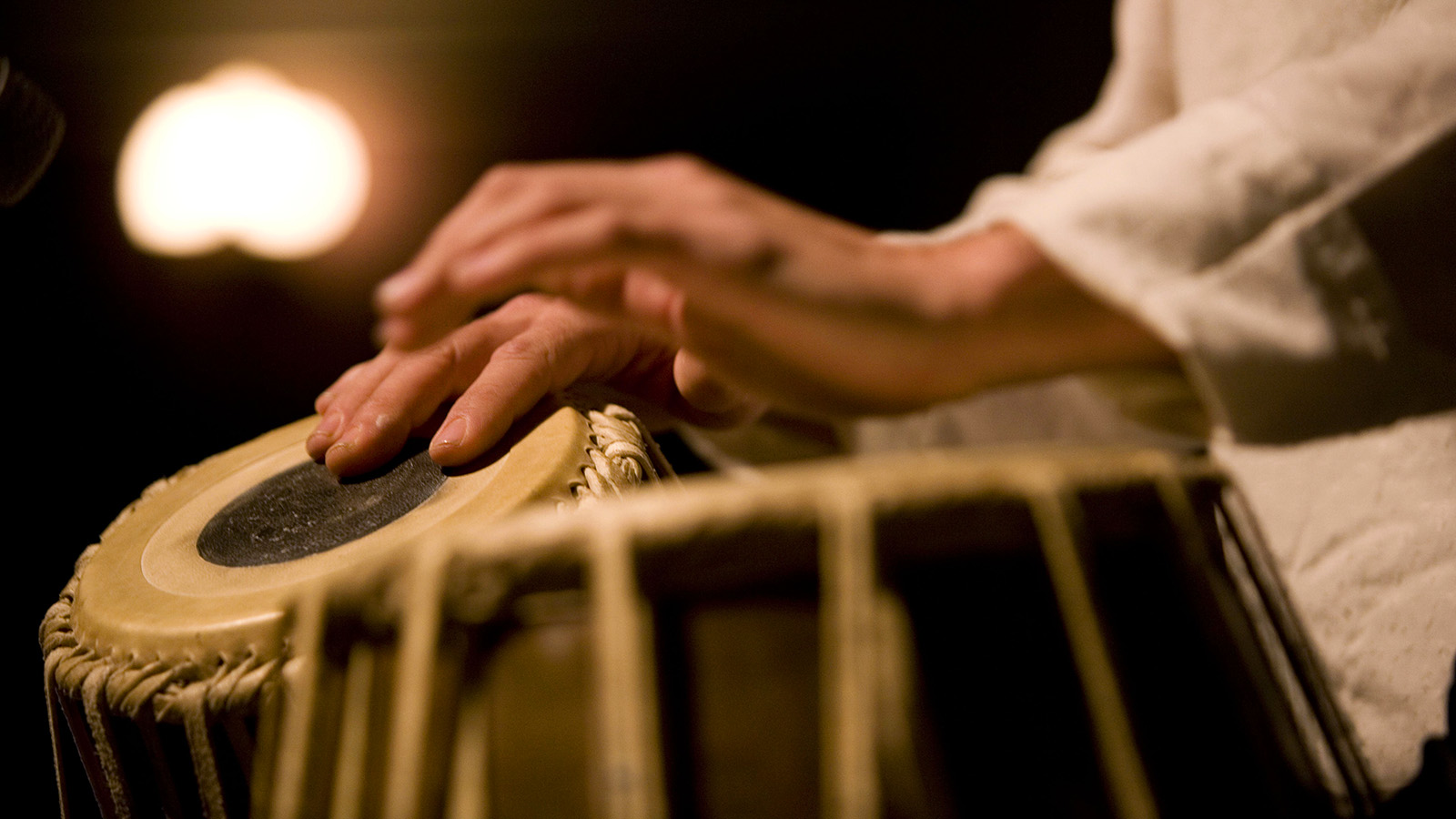In this close-up photograph, a person is intensely focused on playing a set of bongo drums. The individual, wearing a white, long-sleeve cotton top that extends to their wrists, has their hands positioned over the drums, with one hand striking and the other hovering. The hands, cast in a mid-brown hue, bring dynamic energy to the scene. The bongo drums themselves are a light tan or khaki color, featuring a darker slate gray or black circular centerpiece and intricate string netting around their sides, hinting at a handcrafted or ethnic design. Although the hands and drums are captured in slight motion blur, adding to the sense of rhythm and activity, the overall focus remains evocative. The background is a murky blend of black and dark gray, setting a contrasting stage. A bright white light in the upper left corner emits a subtle orange glow, casting a warm, yet mysterious ambiance over the entire composition.